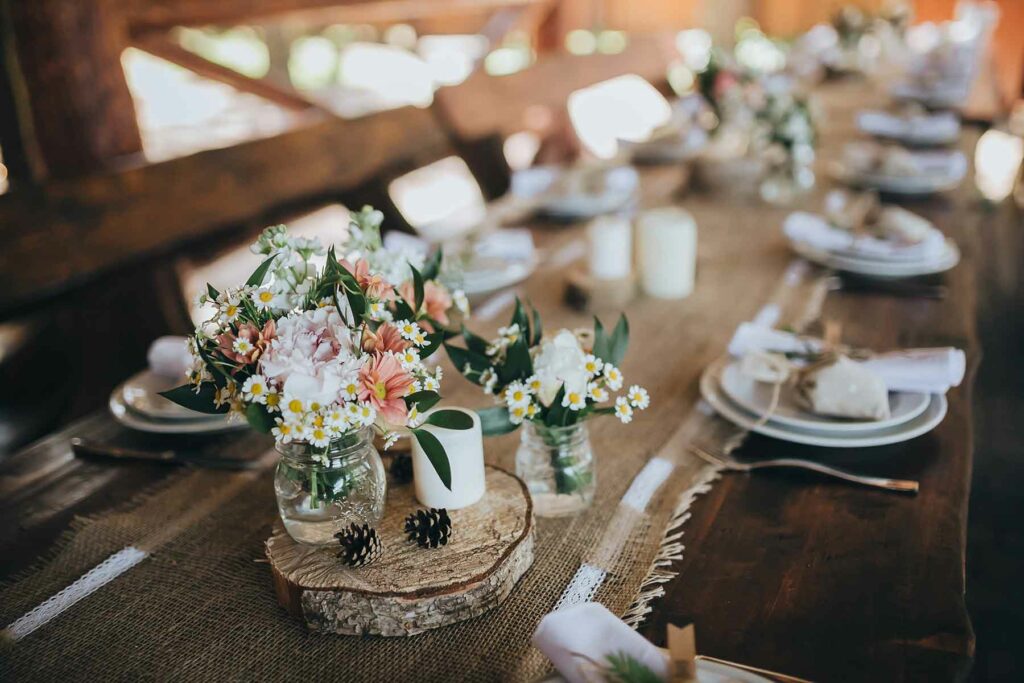The image captures an elegantly rustic table setting, meticulously arranged for a charming outdoor celebration. A burlap table runner elegantly stretches across the table, establishing a natural, earthy foundation. Upon this runner, coasters crafted from cross-sections of tree trunks add a touch of raw woodiness, each adorned with a carefully placed pinecone. Wildflower arrangements, appearing freshly gathered from the surrounding wilderness, inject vibrant splashes of color and life into the scene. Each place setting features a neatly rolled napkin, secured with a strip of brown paper that complements the overall rustic aesthetic. In the blurred distance, rows of similarly adorned settings suggest preparations for a sizable gathering, likely around 20-30 guests, hinting at a festive occasion amidst the natural beauty of the woods.